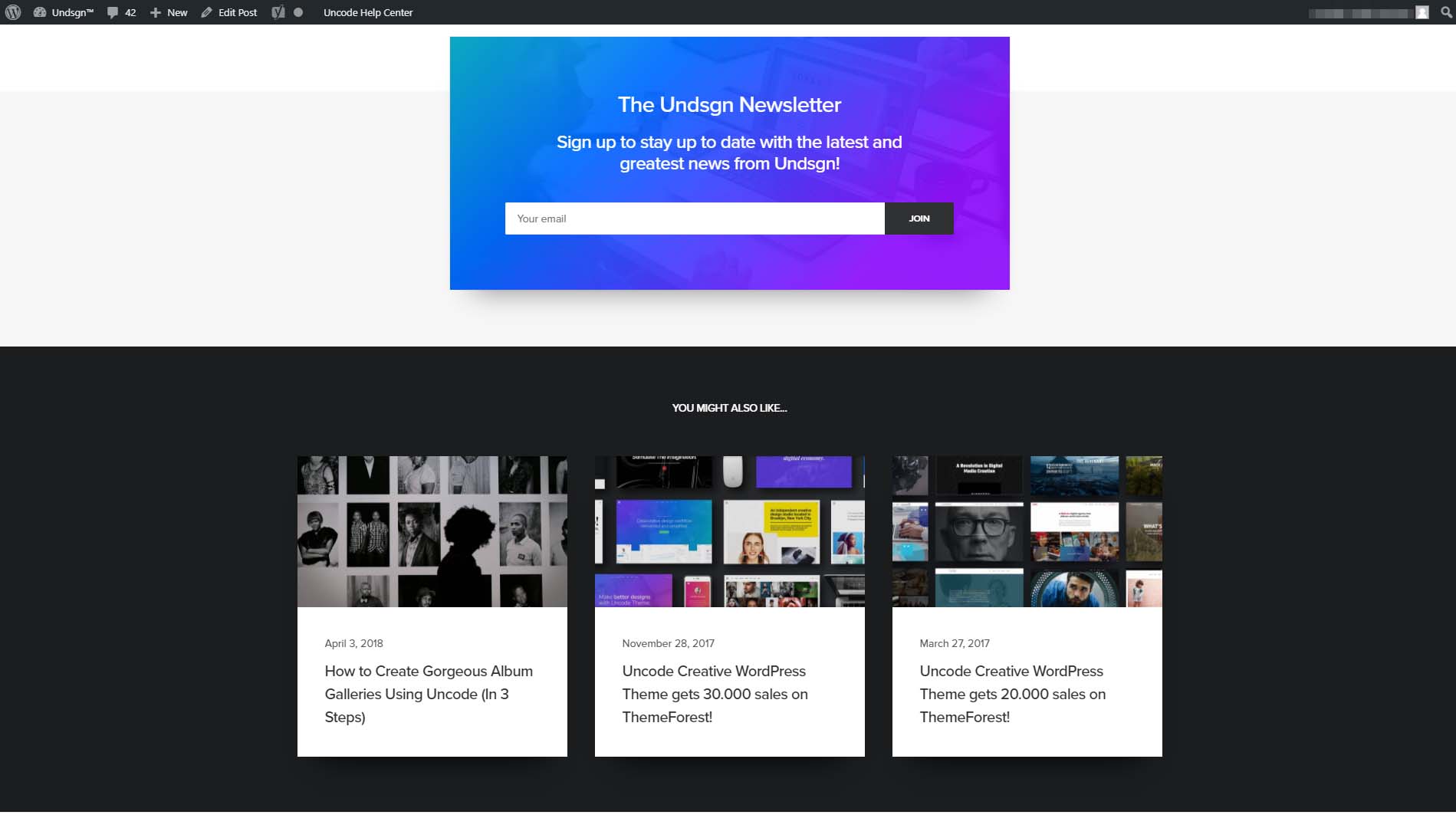At the top of the image, there is a black border with small, blurry text that is difficult to make out. The text appears to be "UNDSGN." Below this, there are several elements including:

- A line of text displaying "42 comments", "new edit post", and "help center".
- A distinctive blue and purple box with the title "UNDSGN Newsletter". The box invites users to "sign up to stay up-to-date with the latest and greatest news from UNDSGN".
- Below the invitation, there is an input field labeled "your email" accompanied by a black button with the text "join".
- Further down, there is a black rectangle containing three white square sections. Each section includes different text:
  - The left section says, "April 3rd, 2018," followed by "How to create gorgeous album galleries using Uncode in three steps".
  - The middle section announces, "Uncode creative WordPress theme gets 30,000 sales on ThemeForest".
  - The right section proclaims, "Uncode creative WordPress theme gets 20,000 sales on ThemeForest".

The overall layout appears to be a combination of promotional and informational content centered around the UNDSGN brand and its Uncode WordPress theme.